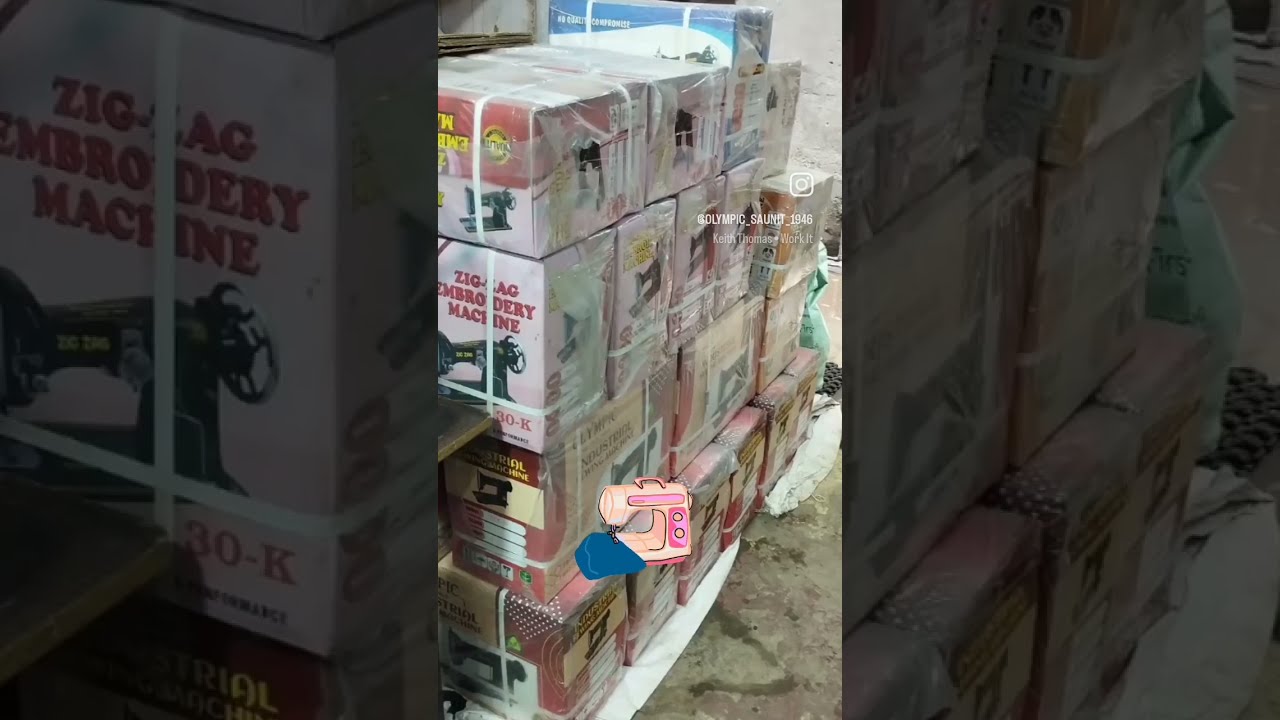The photograph captures a substantial stack of red and white boxes, neatly arranged in a warehouse-like room with a concrete floor, suggesting they are ready for delivery. The boxes form a structure four layers high and about four to five boxes long. Each box is tightly wrapped in plastic with white plastic bands. Prominently, there's a clear, centrally-located drawing of a sewing machine on the front of each box, with the words "zigzag embroidery machine" partially visible in red font on several boxes. Notably, a closer inspection reveals a cartoonish image of a pink sewing machine with its needle area facing left, adorned by a piece of blue material and two knobs on its right side. The photograph, interestingly, consists of three sections: the main image in the center with brighter lighting, and two darker, zoomed-in side images that frame the central picture, emphasizing the boxes' texture and details. Despite some mentions of an outdoor appearance due to the ground's brownish-gray hue resembling dirt or gravel, the setting is definitively inside, illuminated brightly, enhancing the scene's vividness and highlighting an Instagram handle "Olympic_sant_1946" in the upper right corner.